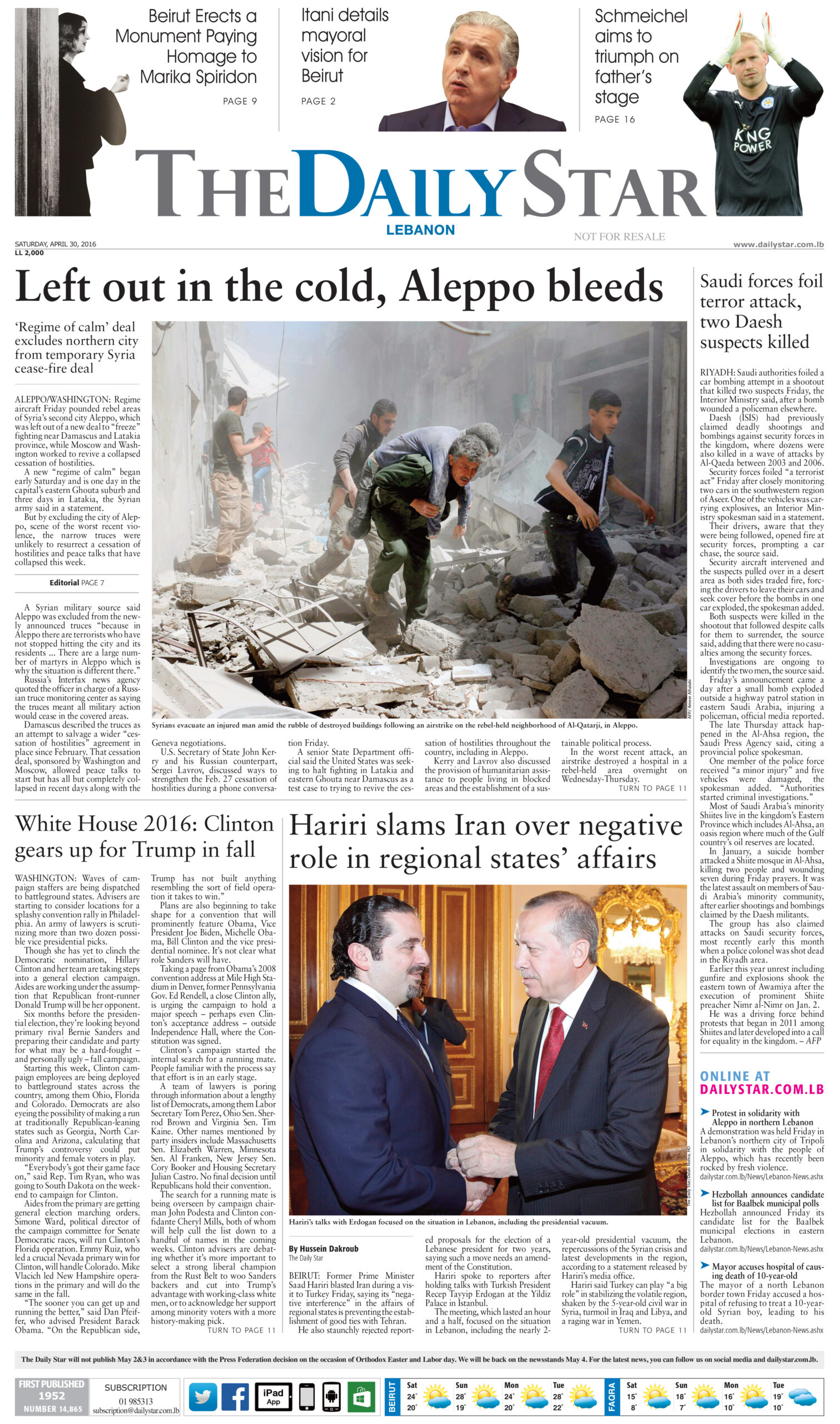This is a screenshot or a scan of a newspaper named "Daily Star Webanon". The newspaper name is prominently displayed at the top, with "Daily" in blue font and "Star Webanon" also in blue.

The top section features three headlines:

1. "Beirut Erects a Monument Paying Homage to Marika Spryden"
2. "Atani Details Mayoral Vision for Beirut"
3. "Schmiel Aims to Triumph on Father's Stage"

Below these headlines is the front page, dominated by the somber main headline: "Left Out in the Cold: Aleppo Bleeds". Accompanying this headline is a heartbreaking photo of a family covered in dust, walking over rubble and broken concrete, symbolizing a major tragedy. In the image, an elderly man is seen carrying an old woman on his back, further amplifying the despair and sorrow depicted.

To the right of this main story, there is an article titled "Saudi Forces Foil Terror Attack: Two Daesh Suspects Killed".

At the bottom of the front page, another headline reads: "White House 2016: Clinton Gears Up for Trump in Fall".